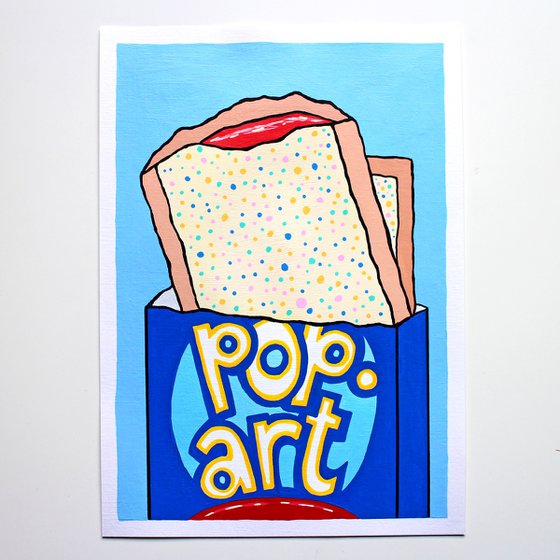The image features a playful, cartoony pop art representation of two strawberry Pop-Tarts emerging from a vertical cardboard box labeled "Pop-Dot-Art." The drawing, which has a light gray background, is rendered on a rectangular piece of white paper. The Pop-Tarts are characterized by a light red base with white frosting speckled with polka dots, and one appears to have a bite taken out, revealing a red filling. The dark navy blue box displays the words "Pop-Dot-Art" in white letters outlined with a darker blue and a yellow shadow, with lighter blue and maroon embellishments. The overall style is deliberately simplistic and reminiscent of a child's crayon or pencil drawing, blending a sense of irony with a charming, low-fi aesthetic.